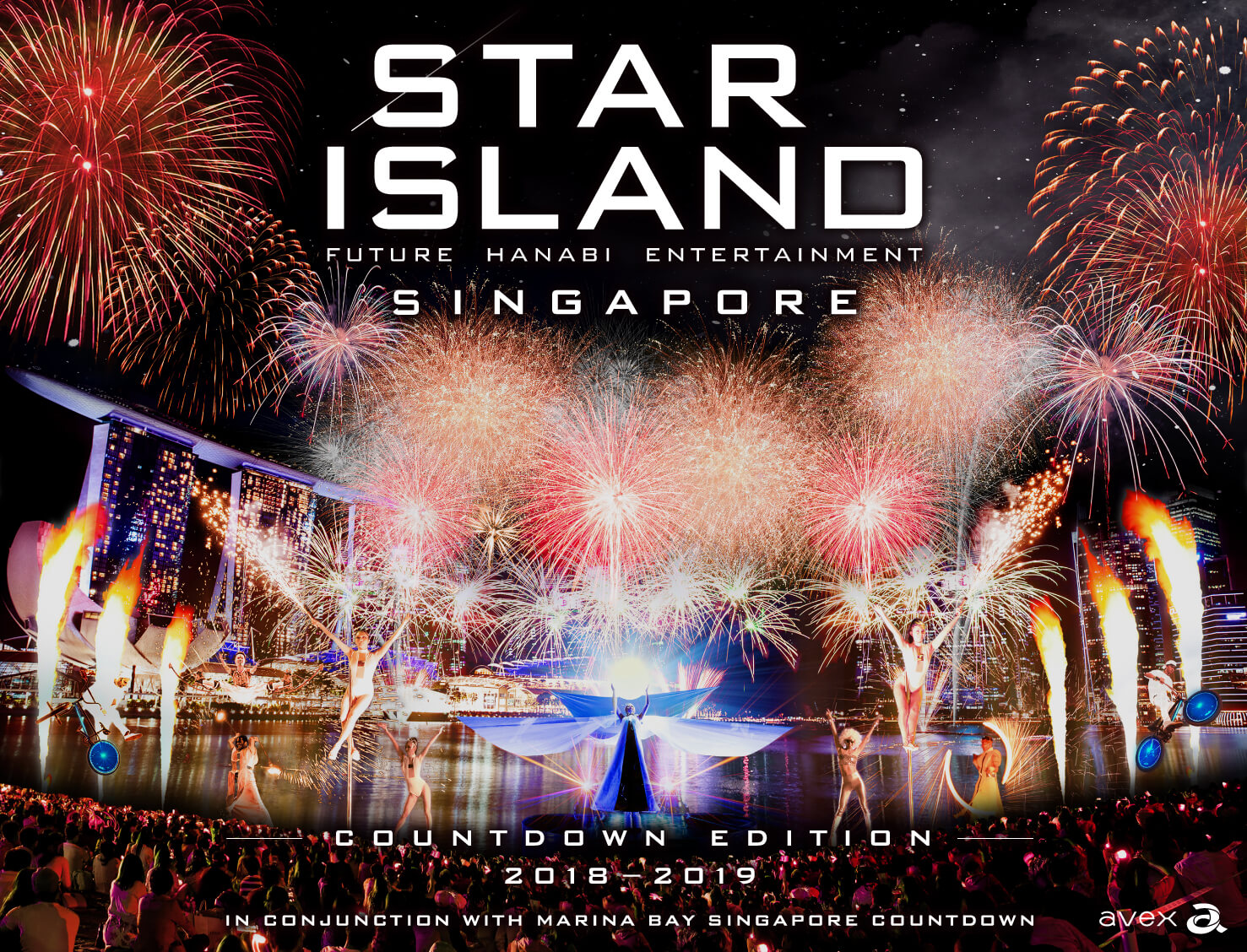The image is a vibrant, full-color poster, seemingly for an outdoor event using artificial lighting at nighttime. Against a night sky backdrop filled with white stars and colorful fireworks, a dynamic scene unfolds. The stage at the bottom teems with activity, featuring an array of performers and dancers holding sparklers. The scene is bustling with small and large figures, with many people in the crowd surrounding the stage, adding to the lively atmosphere. In the background, high-rise resort structures are faintly visible.

Taking center stage at the top of the poster, the text reads in large white capital letters: "star," followed by "island" in slightly smaller capitals. Below this, the text continues in small capital letters: "future Hanabi entertainment, Singapore." Near the bottom, the caption clarifies that this is the "Countdown Edition 2018–2019, in conjunction with Marina Bay Singapore Countdown." To the lower right corner, the company name "AVEX" appears. The poster captures a night sky full of fireworks, energetic performers on stage, and a celebration in full swing, encapsulating the essence of a grand countdown event.